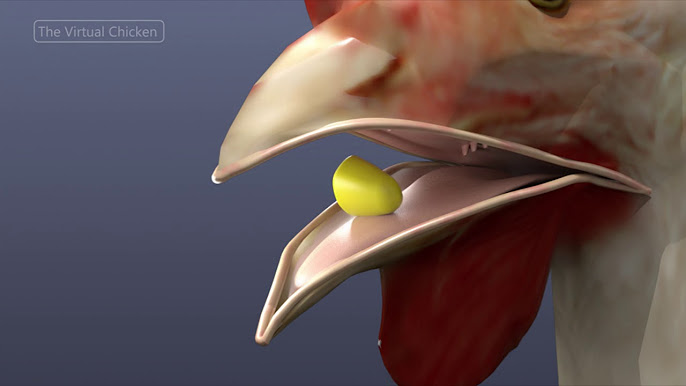This image is a multi-color digital artwork with a horizontally rectangular format and no border. It showcases a close-up view of a chicken's beak, predominantly focusing on the details of the beak and mouth. The background of the image is a grayish color. In the upper left-hand corner, there's text that reads "The Virtual Chicken," enclosed within a light gray-bordered box.

To the right of the text, the primary feature is the chicken's open beak, which is white. Inside the beak, there's a yellow piece of corn resting on the tongue. The mouth is clearly open, revealing the chicken's wattle beneath the beak— a reddish tissue indicative of poultry. The area behind the beak has a marbled appearance, blending white and pinkish hues, reminiscent of meat. The rest of the visible portion of the chicken consists of white feathers, adding to the detailed texture of the image. You can also catch a glimpse of the bottom arc of the chicken's eye, which appears to be brown. The overall image suggests a somewhat low-quality 3D model, with an emphasis on color and texture details.